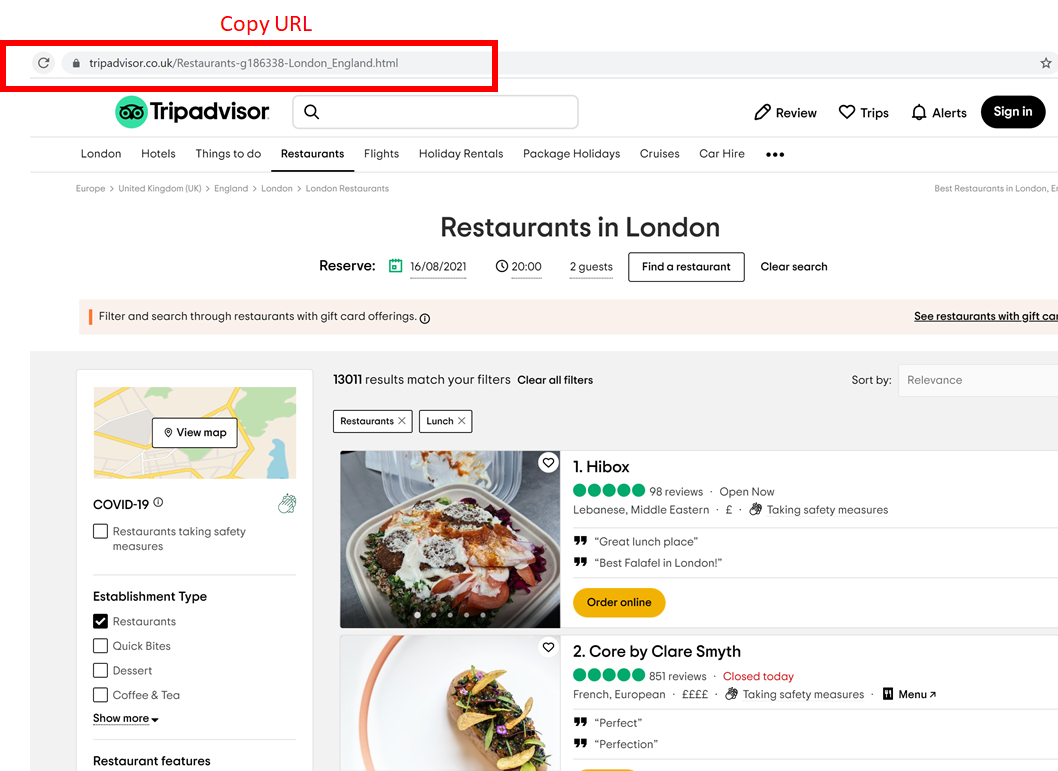The image appears to be a screenshot of a TripAdvisor webpage viewed in a web browser. At the very top of the image, there is a URL bar, with a typed URL outlined by a red box. Above this red box, the text "Copy URL" is displayed. 

Below the URL bar, the TripAdvisor logo and name are prominently featured on the left. Next to the logo is a search box which is currently empty. Moving to the right, there are several icons and labels: a pencil icon labeled "Review," a heart labeled "Trips," a bell labeled "Alerts," and a black, oblong "Sign In" button.

Underneath this interface, a horizontal menu features categories such as "London," "Hotels," "Things to Do," and importantly, "Restaurants," which is highlighted and underlined, indicating it is the current section. Additional menu items include "Flights," "Holiday Rentals," "Package Holidays," "Cruises," "Car Hire," and a three-dot "More" options button.

Further down, separated by a thin gray line, is a section titled "Restaurants in London." This part contains options to reserve a table, with fields to select date parameters, time, and number of guests. A "Find a Restaurant" button, outlined in black, and a "Clear Search" option are also present for refining or resetting the search criteria.